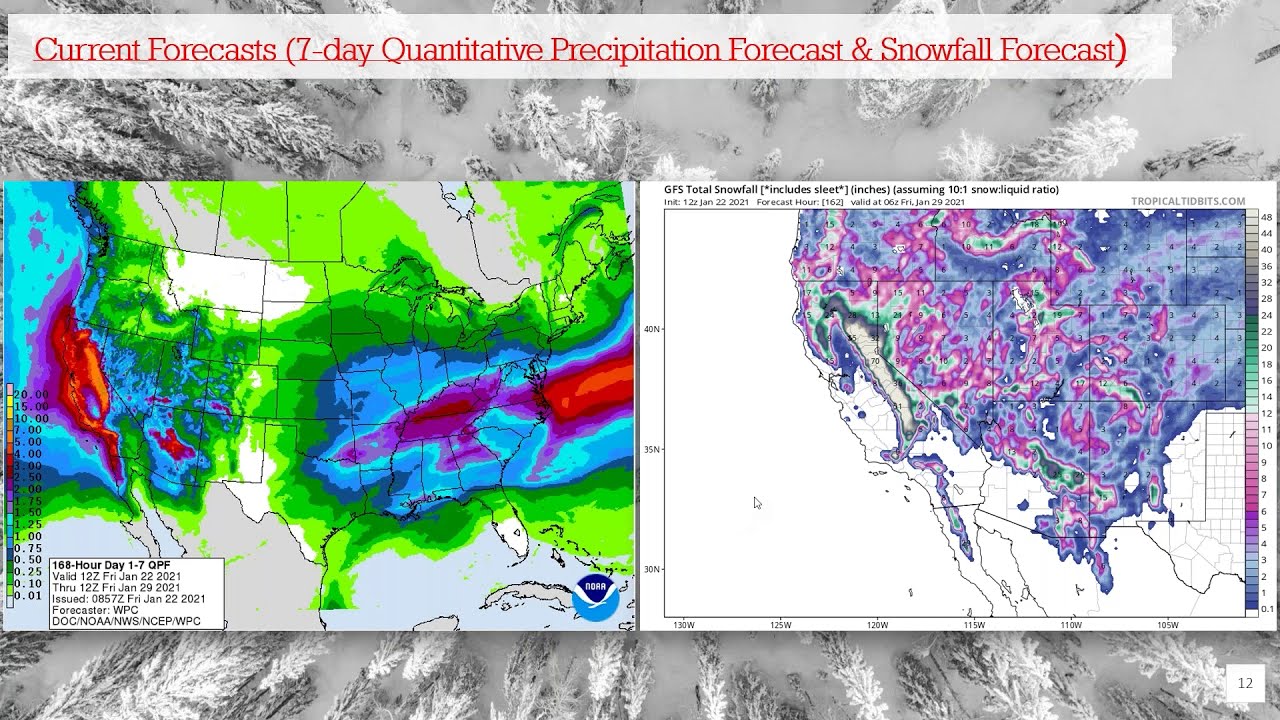The image features two weather maps set against a wintry background resembling a frosty aerial view of snow-covered trees. A small rectangular banner in red text reads "Current Forecasts (7-day Quantitative Precipitation Forecast and Snowfall Forecast)."

The left map displays the entire United States, showing the rainfall totals for a specific day. It is vibrant with colors indicating varying precipitation levels: deep reds over Tennessee and Kentucky, lighter blues surrounding Illinois, Missouri, Georgia, and Ohio, and dark reds extending from northern California to Oregon. Most of the country shows lighter shades of green, except areas like Montana which have no precipitation.

The right map offers a focused view of the western half of the United States, illustrating snowfall ratios. This map also uses dark and light hues of blue and purple to highlight heavy snowfall in states such as Nevada, Colorado, Montana, and Wyoming, while lower California and Arizona remain blank, indicating no snowfall. Additional text in black specifies, "GFS total snowfall includes sleet inches assuming 10:1 snow liquid ratio and 168-hour day 1-7 QPF."